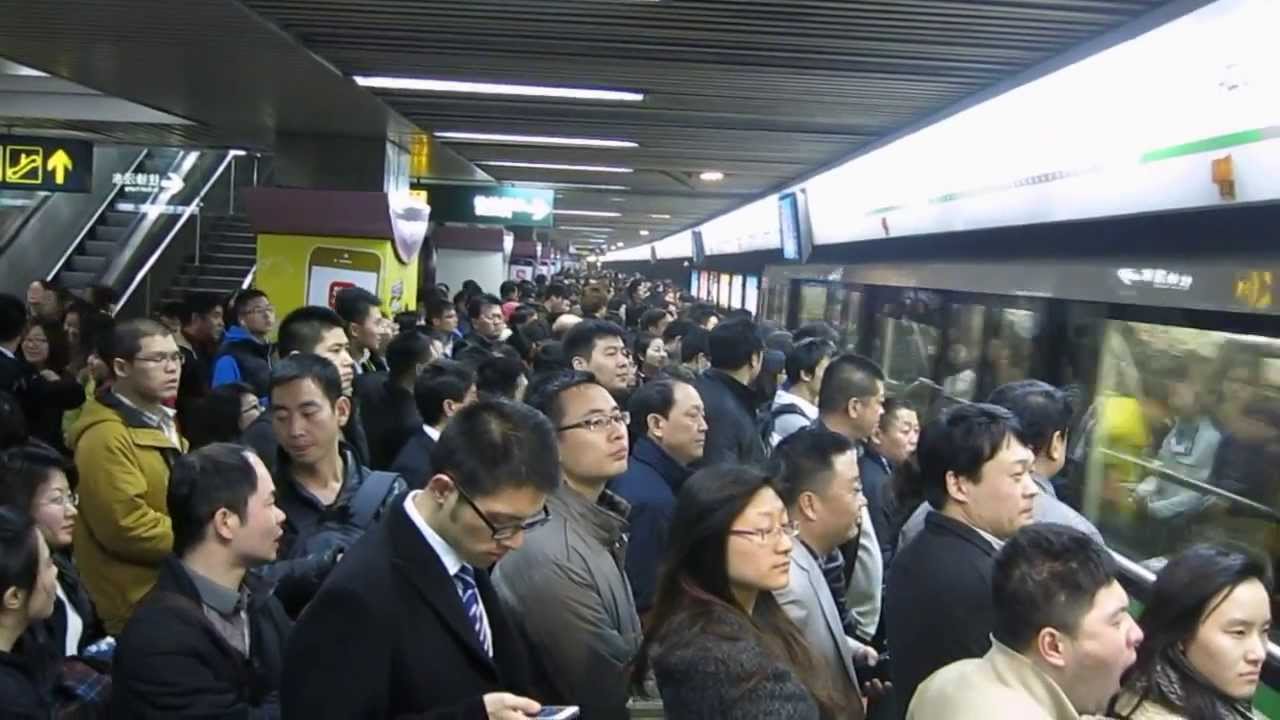The image captures a bustling scene of a crowded subway station, most likely in China, with a diverse group of individuals, majority dressed in business attire, waiting to board a train. The station is packed shoulder to shoulder, evoking a sense of claustrophobia as people jostle for space near the arriving train. The frontmost individuals are so close to the train that their reflections are visible in the windows. Overhead, tube lights illuminate the station, contrasting with the dark gray ceiling above. On the far right, the walls above the train are stark white. Multiple signs with Asian characters and arrows are visible throughout, including one directing people towards a set of stairs leading upwards, while an escalator is seen on the left descending into the subway area. The image, slightly blurred, captures the dynamic and hectic nature of a typical metro commute in a densely populated urban area.